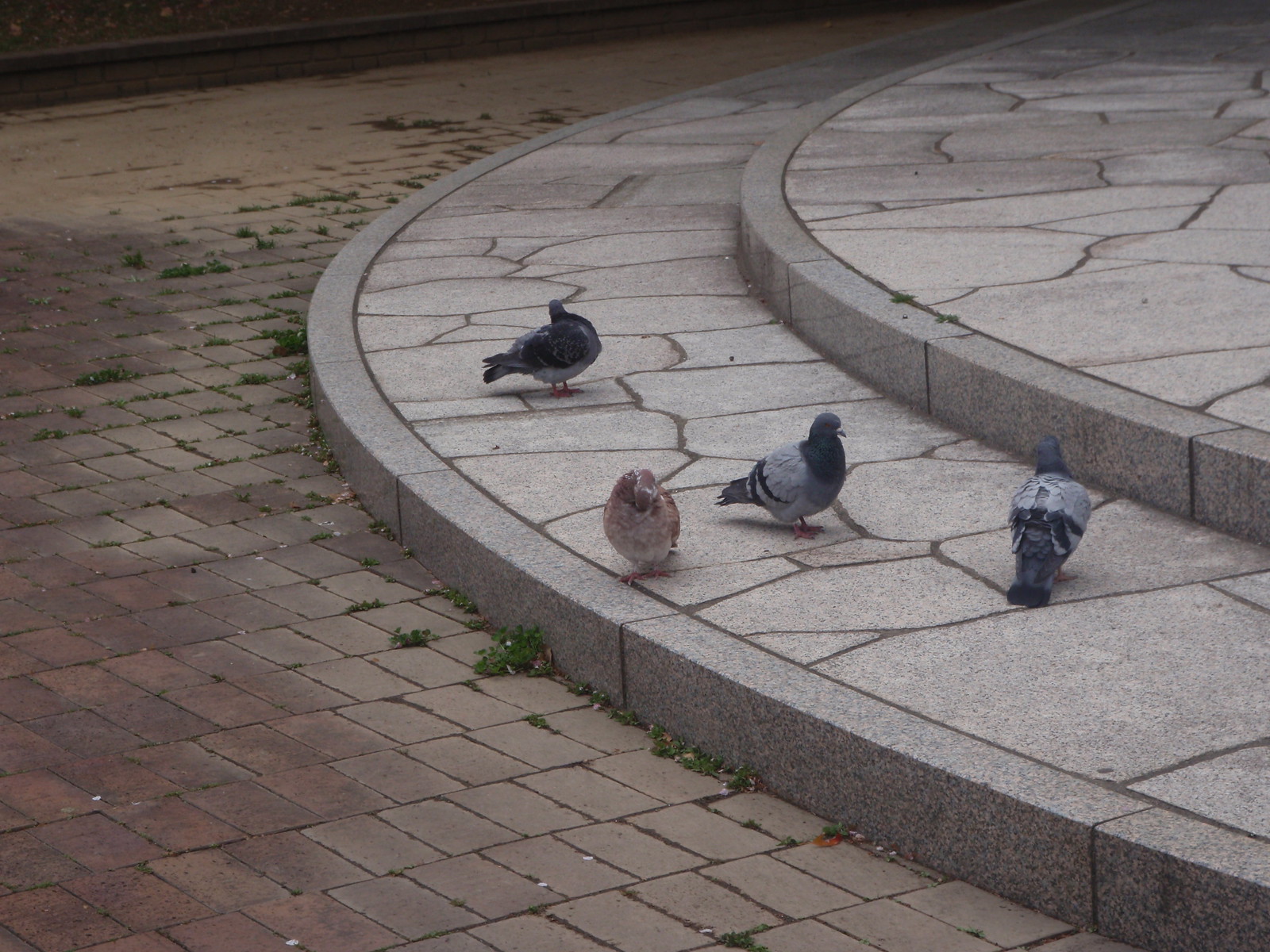This photograph seems to have been taken outdoors at night, capturing a circular stone structure possibly surrounding a fountain, though the actual fountain is not visible. The prominent feature on the right side of the image is two giant curved steps, made up of irregularly shaped, light gray and dark gray flat rocks. Four pigeons are scattered on the lower step. These pigeons exhibit diverse color patterns: one is all black, another is light gray with black markings, a third has a black head with a gray body and blue lines, and the fourth features an unusual rosy hue with beige and hints of pink. On the left side, the scene transitions into an old, weathered brick pathway with some grass and weeds poking through the gaps, adding a touch of nature's reclamation to the setting. The pigeons, with their wings folded in, create the central focus of this nocturnal outdoor photograph.